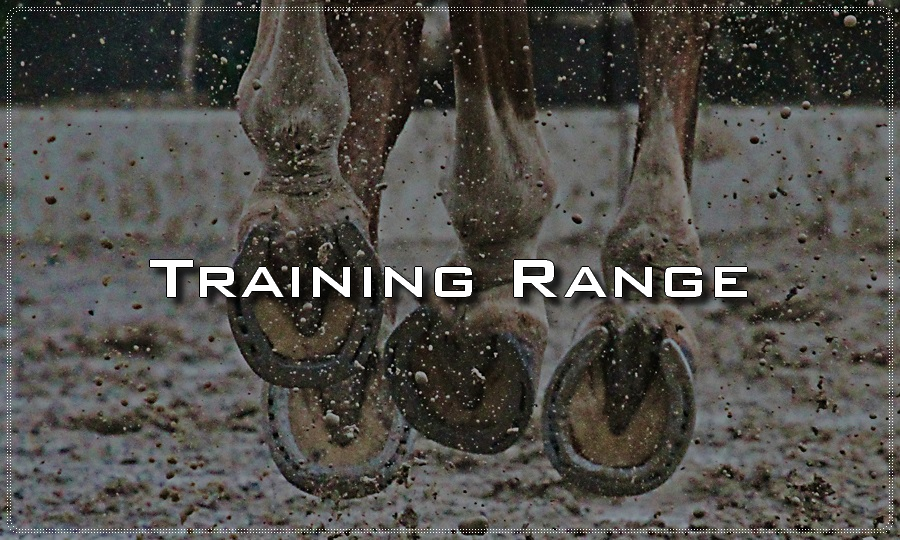This photograph captures a dynamic close-up of a horse's hooves in mid-run, with all four hooves off the ground, encapsulating the power and motion of its stride. Each hoof is fitted with a well-maintained, silver-colored horseshoe that gleams despite the surrounding dirt and mud being kicked up by the horse's movement. The horse's legs are a medium brown with creamish white around the ankles, adding contrast to the scene dominated by a muddy terrain, emphasizing the vigorous action taking place. Overlaid in bold white capital letters in the center of the image are the words "Training Range." The entire image exudes energy and motion, framed by a subtle, small white dotted border that suggests it might have been cropped from a web page. The background is a blend of gray and white, adding to the rugged training atmosphere.